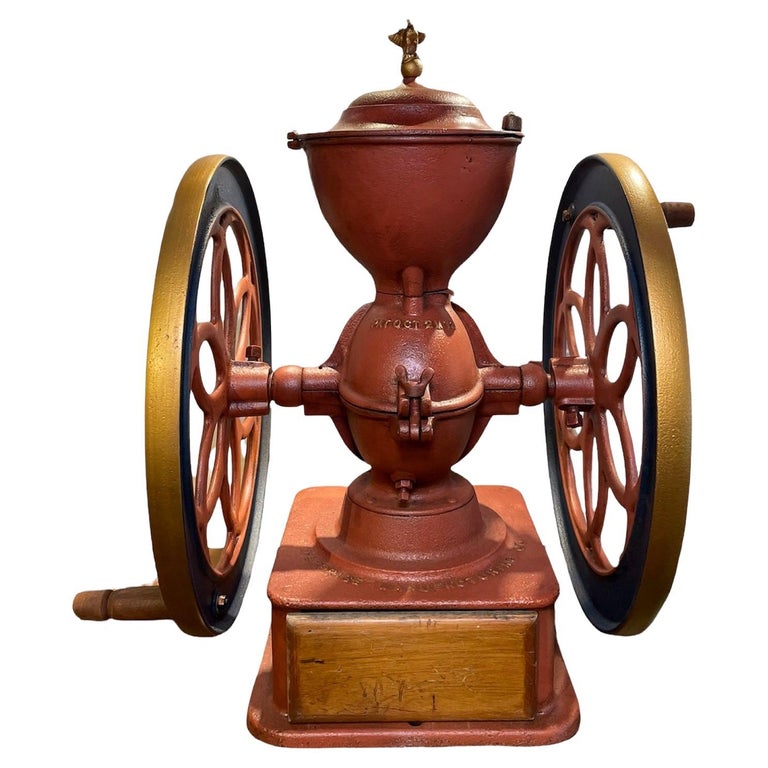The image depicts a butter churner-type contraption with a wooden base, standing on a pedestal that features a wooden plate on the front. At the center of the apparatus, there is an egg-shaped container that is copperish in color with gold accents. This container is connected to two intricately designed wheels, each of which is adorned with a flower pattern made of metal and equipped with a knob for turning. The top of the container resembles an urn, complete with a lid that features a small, designed handle for lifting. The whole structure gives the appearance of being crafted from a material that suggests a rusty, clay-brick hue.